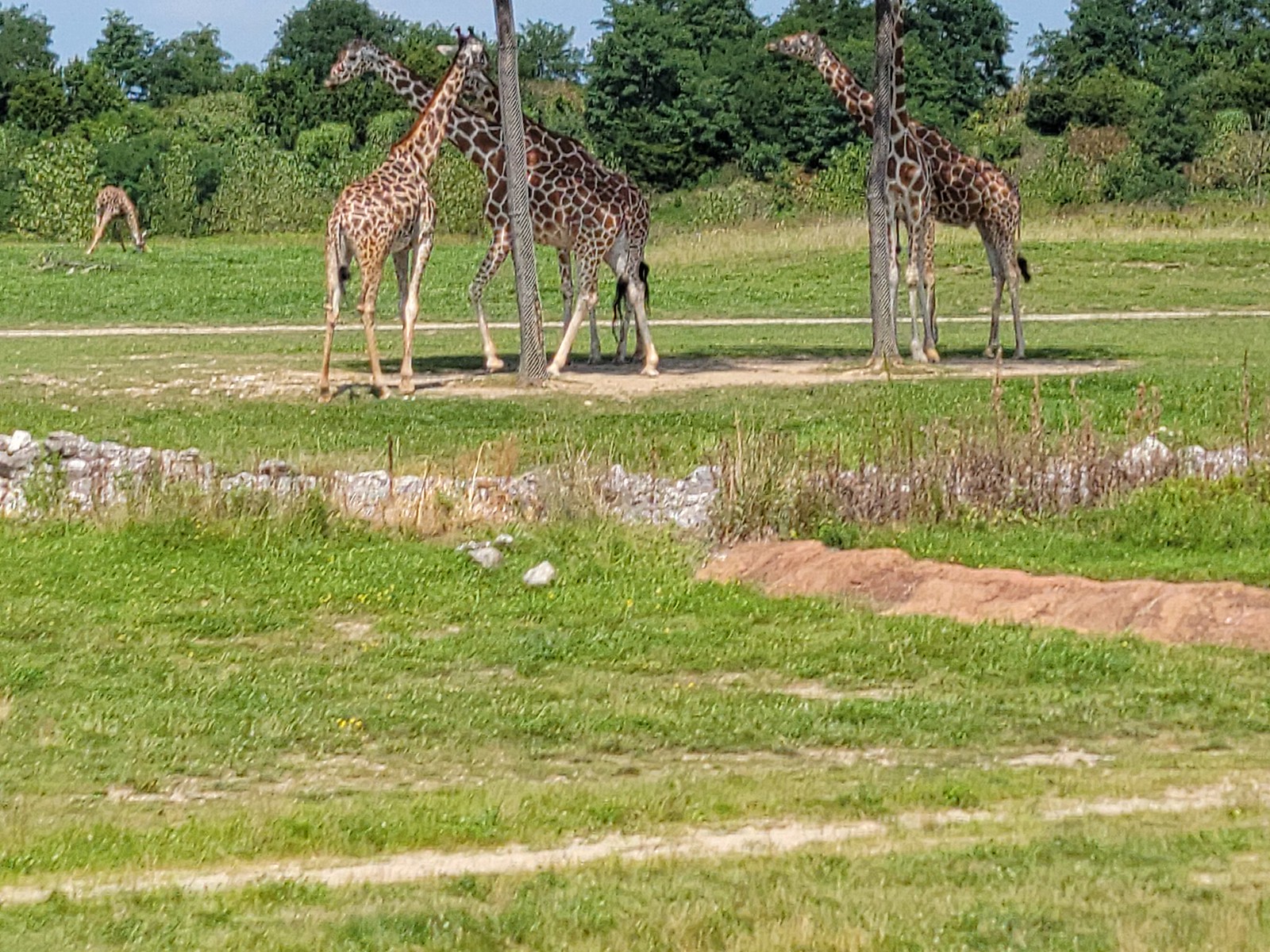The photograph captures a serene scene within a giraffe enclosure, framed by a backdrop of blue sky and dense green trees, ranging in hues from hunter to forest green, with lighter green shrubs interspersed. In the middle of a large, partially grassy field with patches of dried grass and dirt, stand four giraffes. Their distinctive coats feature brown spots and white lines, though one giraffe's spots are notably lighter, a caramel or reddish brown. These gentle giants stand peacefully, three clustered beneath the shade of two slender, greenish-barked trees, their positions suggesting a moment of rest and tranquility. Two face left while one faces right, highlighting their calm demeanor. In the distance to the left, a fourth giraffe is seen kneeling with its legs spread apart, its head bent down, grazing on the grass. The harmonious blend of natural elements and the giraffes' placid presence creates a picturesque and detailed snapshot of wildlife in their habitat.